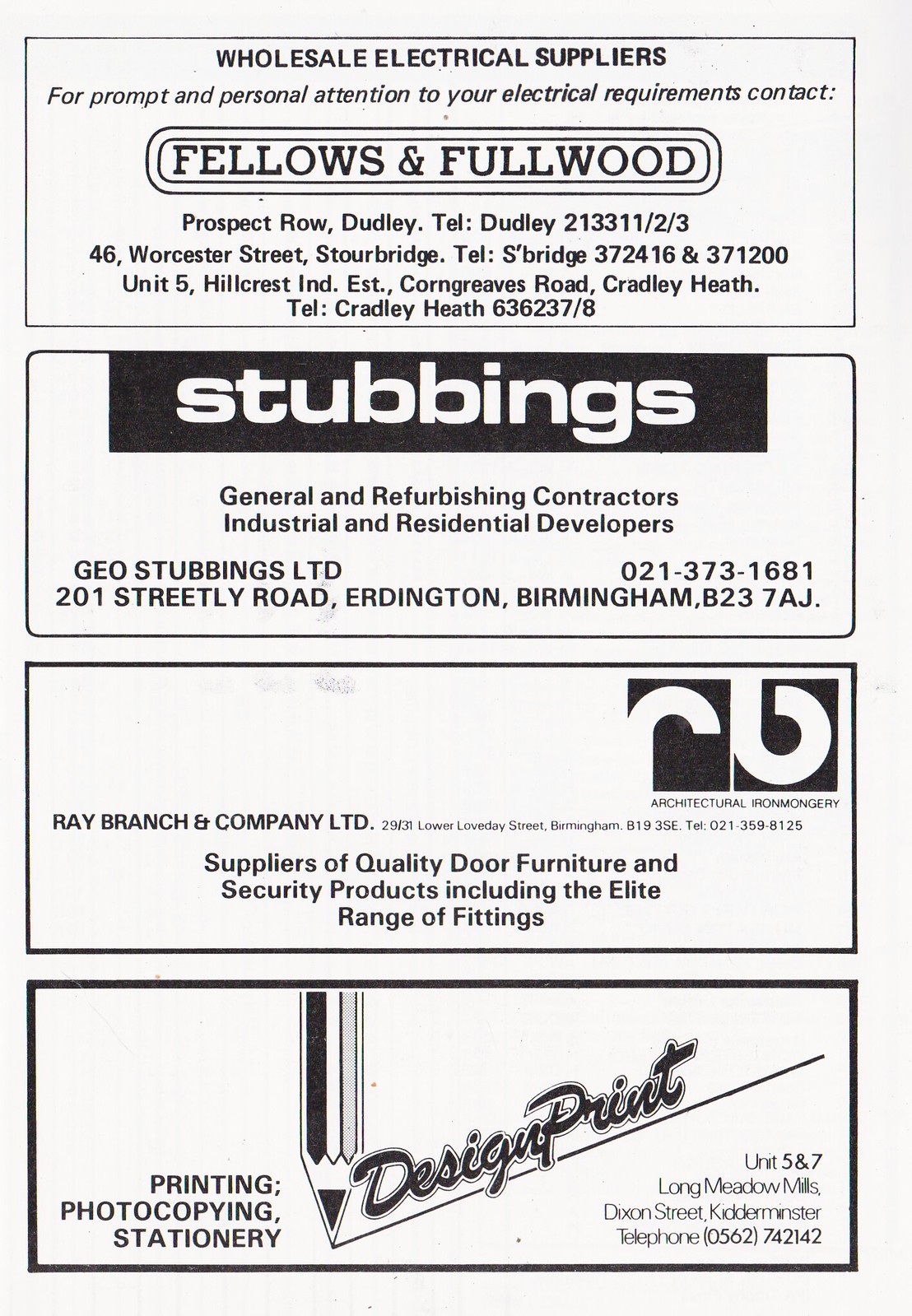This detailed black-and-white image from a newspaper features multiple rectangular advertisements for various companies. The top rectangle advertises wholesale electrical suppliers, promoting prompt and personal attention to electrical requirements. It lists contact details for Fellows and Fullwood at Prospect Road, Dudley, with the phone numbers Dudley 213311/2/3, Worcestershire Street, Stourbridge at S-Bridge 372416 and 371200, and Unit 5 Hillcrest, Ind Est, CornGreaves Road, Cradley Heath at 636237/8.

The second rectangle promotes Stubbings General and Refurbishing Contractors, specializing in industrial and residential development. The contact information provided is GEO Stubbings Ltd, 201 Streetly Road, Erdington, Birmingham, B23 7AJ, with the telephone number 021-373-1681.

The third rectangle is for Ray Branch and Company Ltd, suppliers of quality door furniture and security products, including the elite range of fittings. The contact address is 29-31 Lower Loveday Street, Birmingham, B19 3SE, and the telephone number is 021-359-8125.

The final rectangle highlights design and print services, including printing, photocopying, and stationery. A pencil sketch decorates this ad, which lists Units 5 and 7, Long Metal Mills, Dixon Street, Kidderminster, with the telephone number 0562 742142.